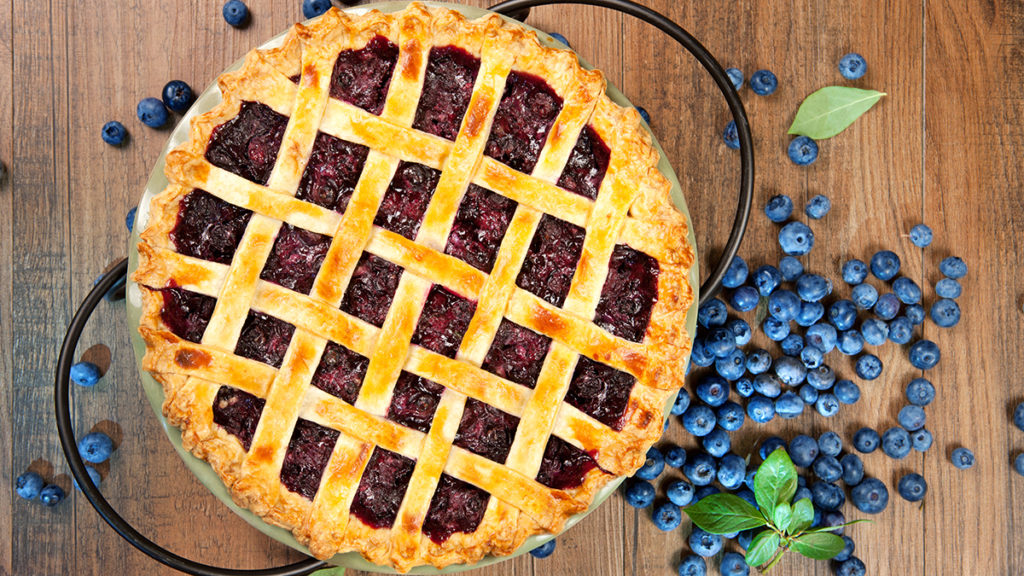This horizontal rectangular image showcases a freshly baked berry pie, likely blueberry, characterized by a golden brown lattice crust that reveals a reddish berry filling. The pie, nestled in a metal pie tin, sits on a black wire pie stand. The rustic setting is enhanced by a dark brown wood-grained tabletop, where fresh blueberries and scattered green leaves, possibly mint, add a burst of color to the scene. The meticulously scalloped edges of the crust and the lattice pattern highlight the pie's homemade appeal, while the blueberries are distributed primarily to the right side of the pie, with a few more scattered on the left, providing a sense of abundance and freshness.